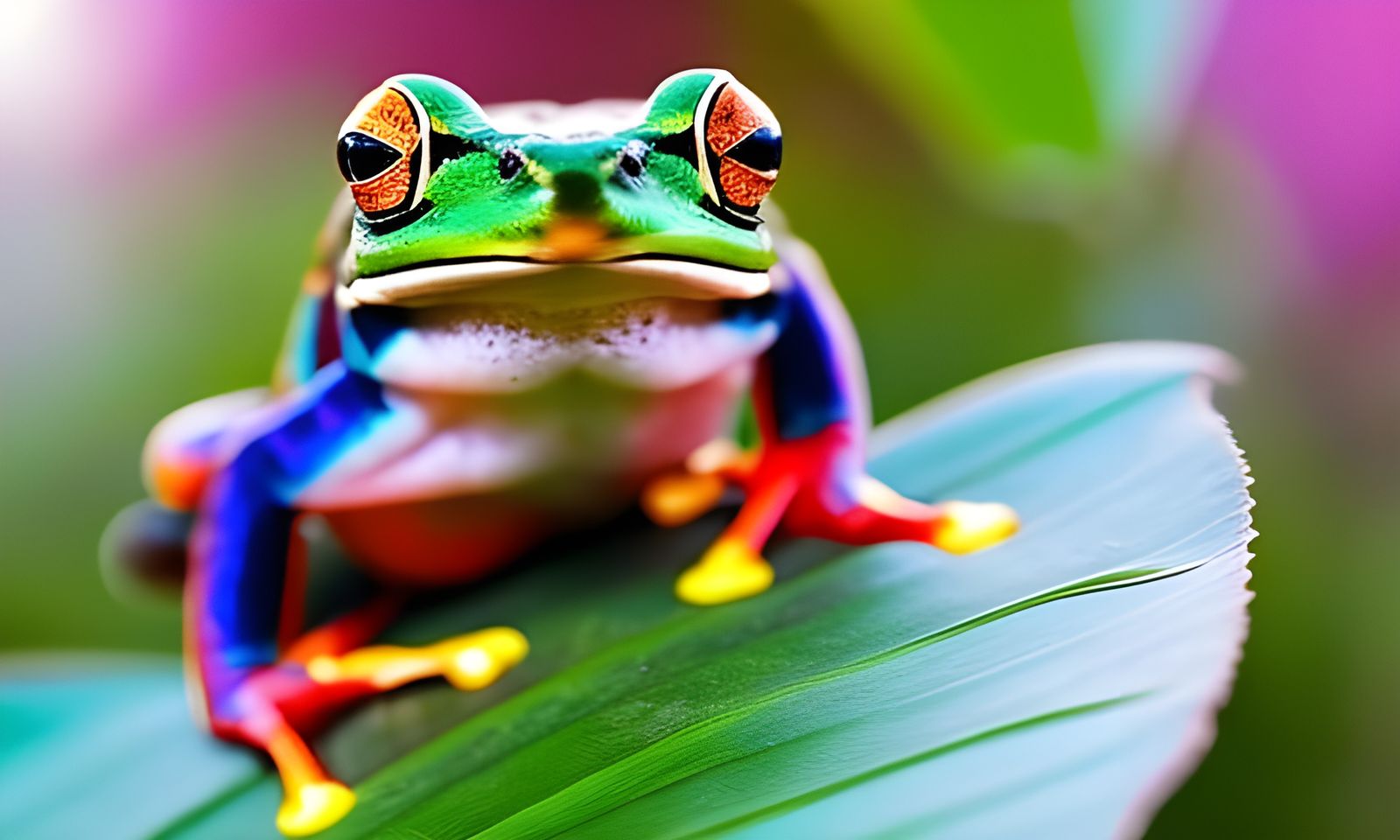In this close-up image, a vividly colorful frog is perched on a large, shiny green leaf. The frog faces directly towards the camera, its bright green face featuring distinctive black stripes near its orangish eyes with black pupils. Below its head, the underside of its chin is mostly white, blending into a blue area that extends to its front legs. The frog's arms are a striking combination of blue, red, and yellow, with its hands appearing orangish-red and its large, yellow fingers ending in round, suction cup-like tips. The chest of the frog is white, while the rest of its body remains out of sight due to the angle. In the backdrop, there are unfocused green and magenta hues, suggesting the presence of other plants or flowers. The leaf beneath the frog transitions from green to blue, adding to the vibrant palette of the scene.